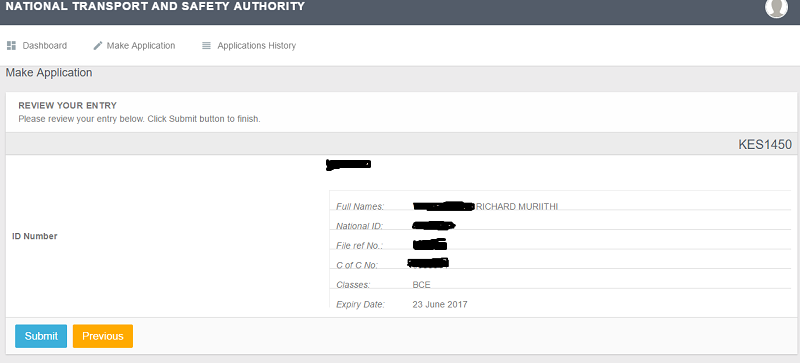The image depicts a web page for the National Transport and Safety Authority. At the top of the page, there is a gray header bar displaying the organization's name in white text. To the right of this header bar, there is a circular profile icon.

The main background of the page is white, showcasing a dashboard layout. In the left-hand section, written in gray, are two clickable options: "Make Application" accompanied by a pencil icon, and "Application History" next to a gray square box.

Below the main header, a subsection titled "Make Application" is also in a gray header bar. This is followed by a white area where instructions are provided in black text, reading: "Review your entry. Please review your entry below. Click submit button to finish."

Further down, another gray header bar prominently displays "KES 1450," indicating a fee or cost. Below this header, there is a white input box labeled "ID Number." The section also includes fields for "Full Names," where the name "Richard Murtithi" is visible, although partially blurred. The national ID number and file reference number (CFC number) have been redacted for privacy. Another field, labeled "Classes," shows the value "BCE," and the "Expiry Date" is listed as "June 23, 2017."